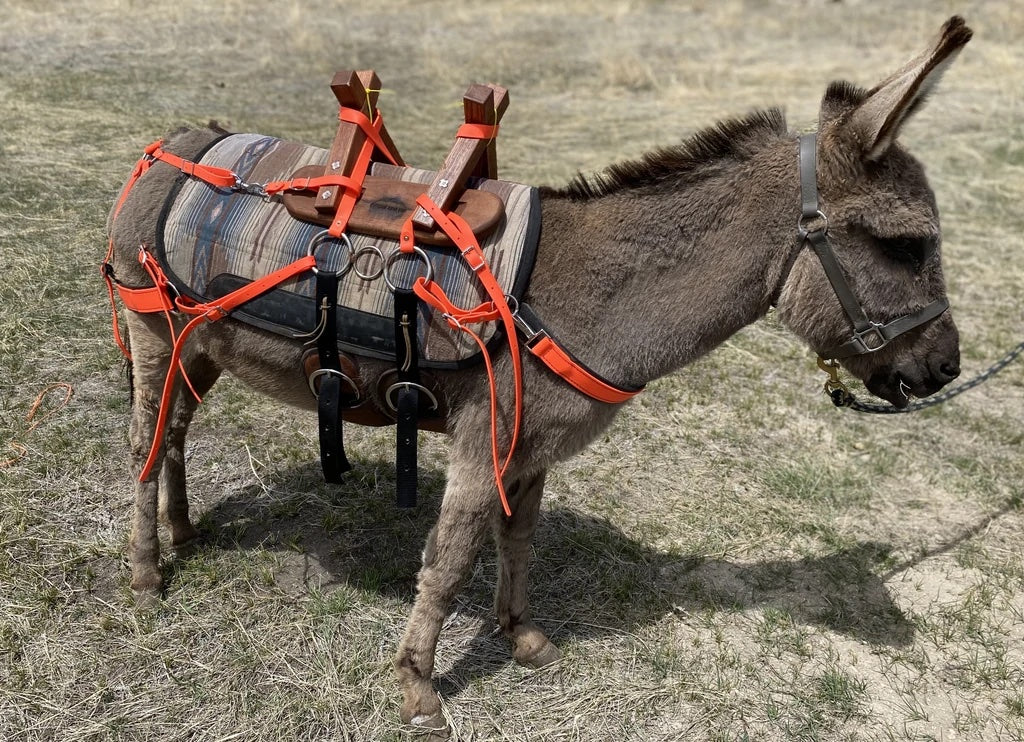The image features a sturdy donkey with brown fur and a black mane, complemented by upright ears with black tufts. This fine-looking fellow is standing on a mixed terrain of green and yellow grass interspersed with tan and brown patches of dirt and sand. The background is filled with a blend of grass, hay, and sticks, adding a natural rustic texture.

The donkey is equipped with a detailed lead bridle, which includes a black leather mouthpiece and a gray and white rope attached to a gold hook on its gray face harness. On his back, there's a red saddle adorned with blue and gray stripes, secured by black leather straps and silver circles. Over the saddle rests a wooden casing, likely used for carrying supplies. The saddle is also supported by intricate harnesses, featuring wooden X-shaped structures and an array of orange webbed ropes that secure the various parts together, wrapping around both the front and rear of the donkey.

Additionally, the donkey boasts a secondary baggage carrier, situated on a blanket to prevent irritation. The entire harness system is fastened with silver hoops and includes visible cinch straps to ensure everything is held tightly in place. The detailed setup of the harness system highlights the donkey's role as a pack animal, prepared for transporting goods. Despite his readiness, the donkey appears to be patiently awaiting further instruction.